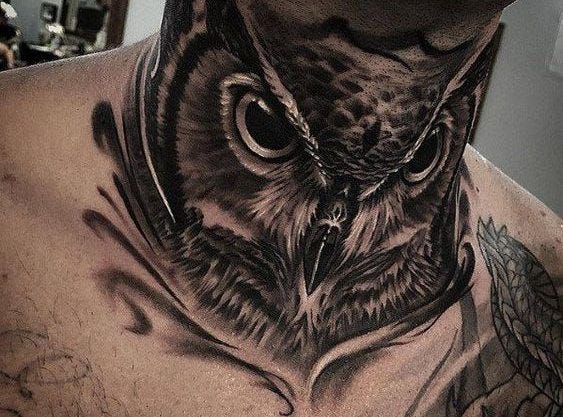The photograph captures a man's neck, shoulders, and a hint of his chest, focusing on an intricate and realistic black-and-white owl tattoo that envelops his neck and wraps around the side. The owl, staring intensely towards the camera, dominates the image with its almost 3D appearance. The tattoo exhibits a semi-healed state, suggesting it may have been completed over multiple sessions due to the lack of redness or bruising. Additional tattoos are partially visible on his left shoulder and right pectoral, including some green ink, though they are not clear due to the image's framing. The man's skin is a tannish peach color, and the background features a white wall, a wooden-trimmed entryway, and what appears to be a mirror with a blurry reflection, indicating the setting is likely a tattoo parlor.